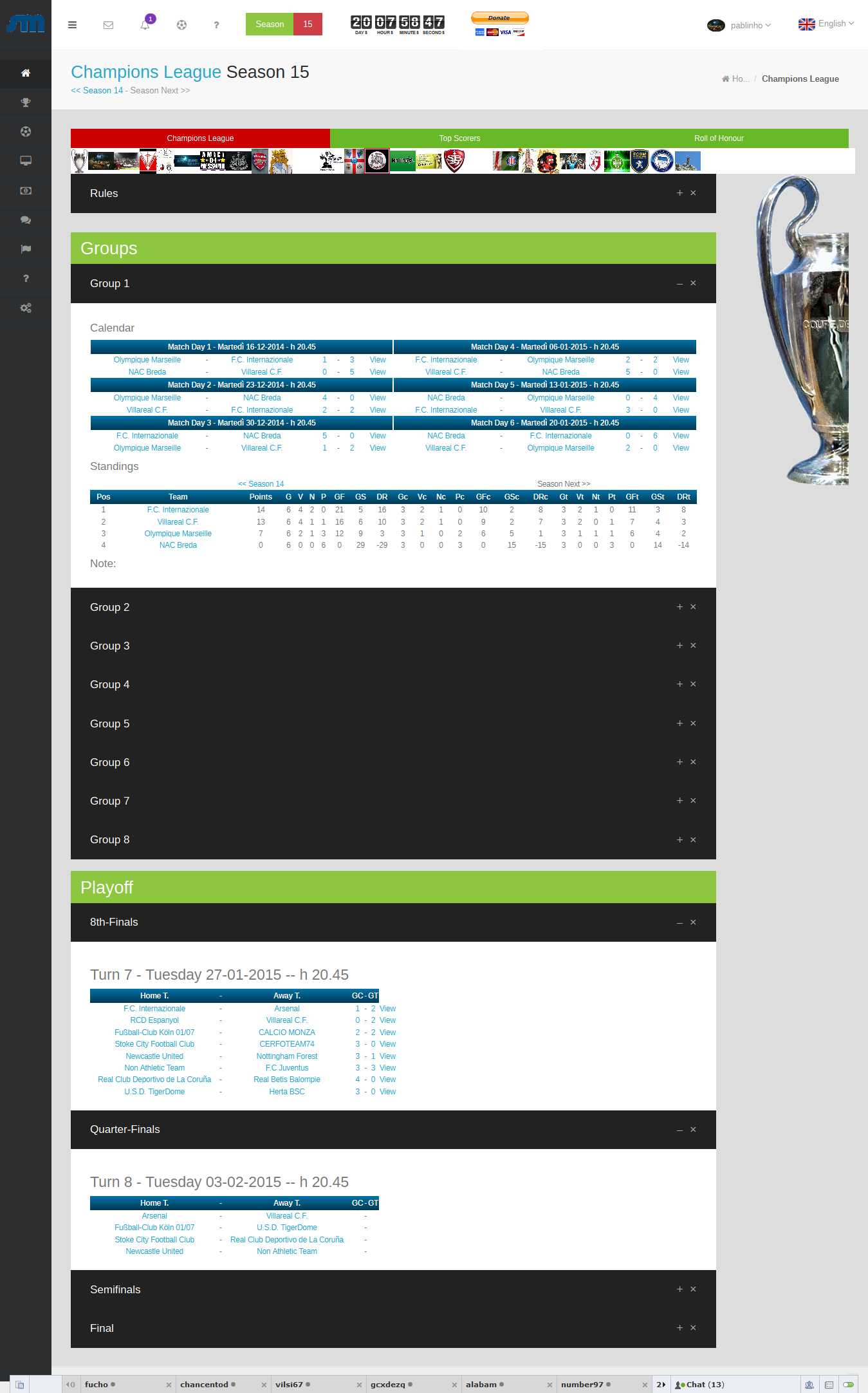Screenshot of a statistics dashboard detailing the Champions League Season 15. At the top left corner, the title "Champions League Season 15" is prominently displayed. Directly beneath it, there is a section titled "Groups" with a subheading of "Group 1." Adjacent to it, the label "Calendar" is visible. The remainder of the text in this area appears to be quite small and difficult to discern. Below this section, a chart is partially visible. Alongside, there are references to additional group names, ranging from Group 2 to Group 8. Above these group names, the text reads "Playoff Turn 7, Tuesday 27-01-2015 H20:45 20.45," indicating a specific match event. At the very bottom of the image, there is a mention of "Turn 8," likely referring to another phase or round in the competition.